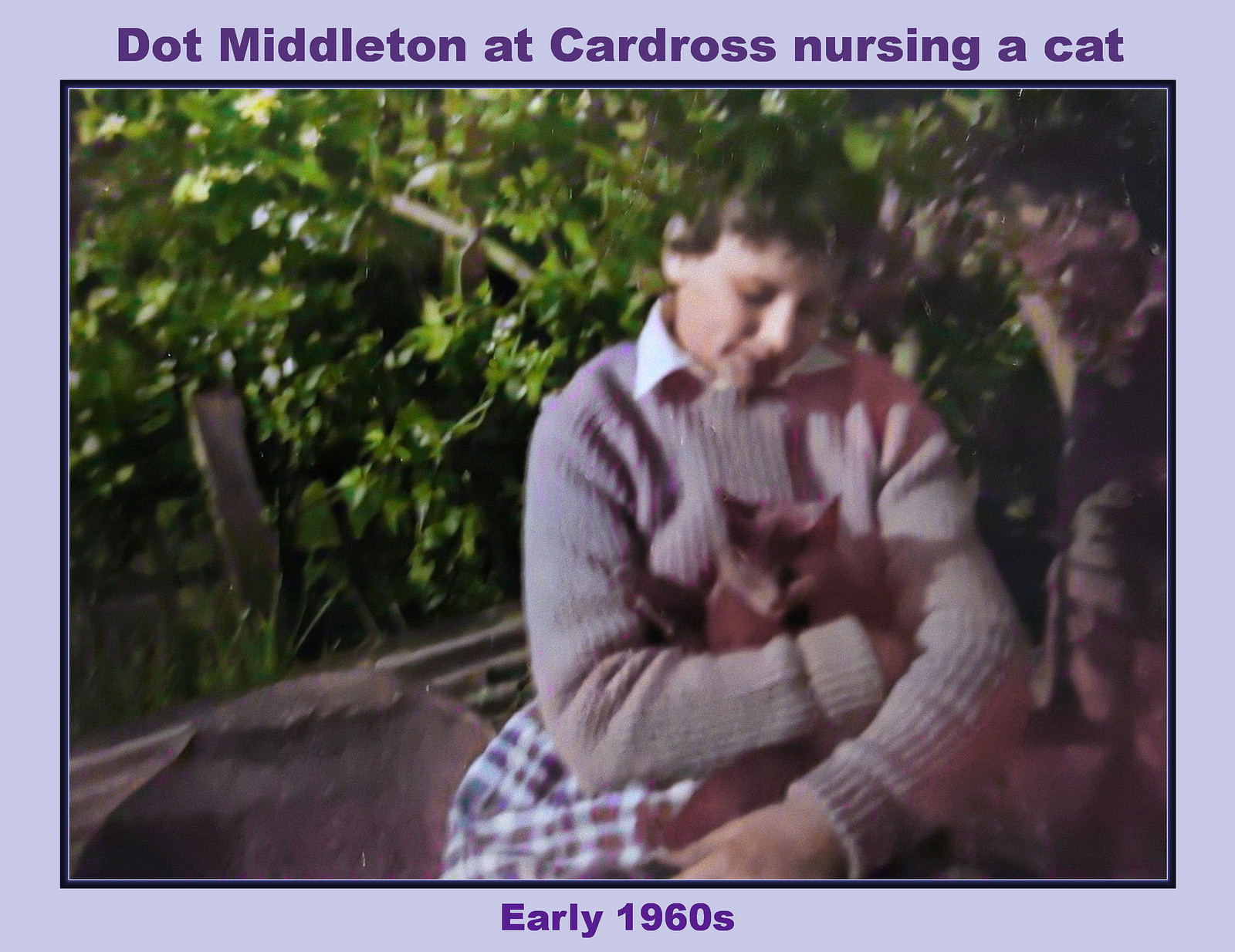In this outdoor photograph from the early 1960s, a young girl named Dot Middleton is seated, nursing a gray short-haired cat in her lap. Dot has a pixie haircut with dark brown hair and is dressed in a gray sweater layered over a white-collared shirt. She wears a pleated skirt in shades of blue, white, and black. The scene features lush foliage with tree branches and leaves in the background, as well as a small wall or cement structure behind her. The image is framed in a light purple-lavender frame, with the words "Dot Middleton at Cardross Nursing a Cat" inscribed in darker purple at the top and "Early 1960s" at the bottom.